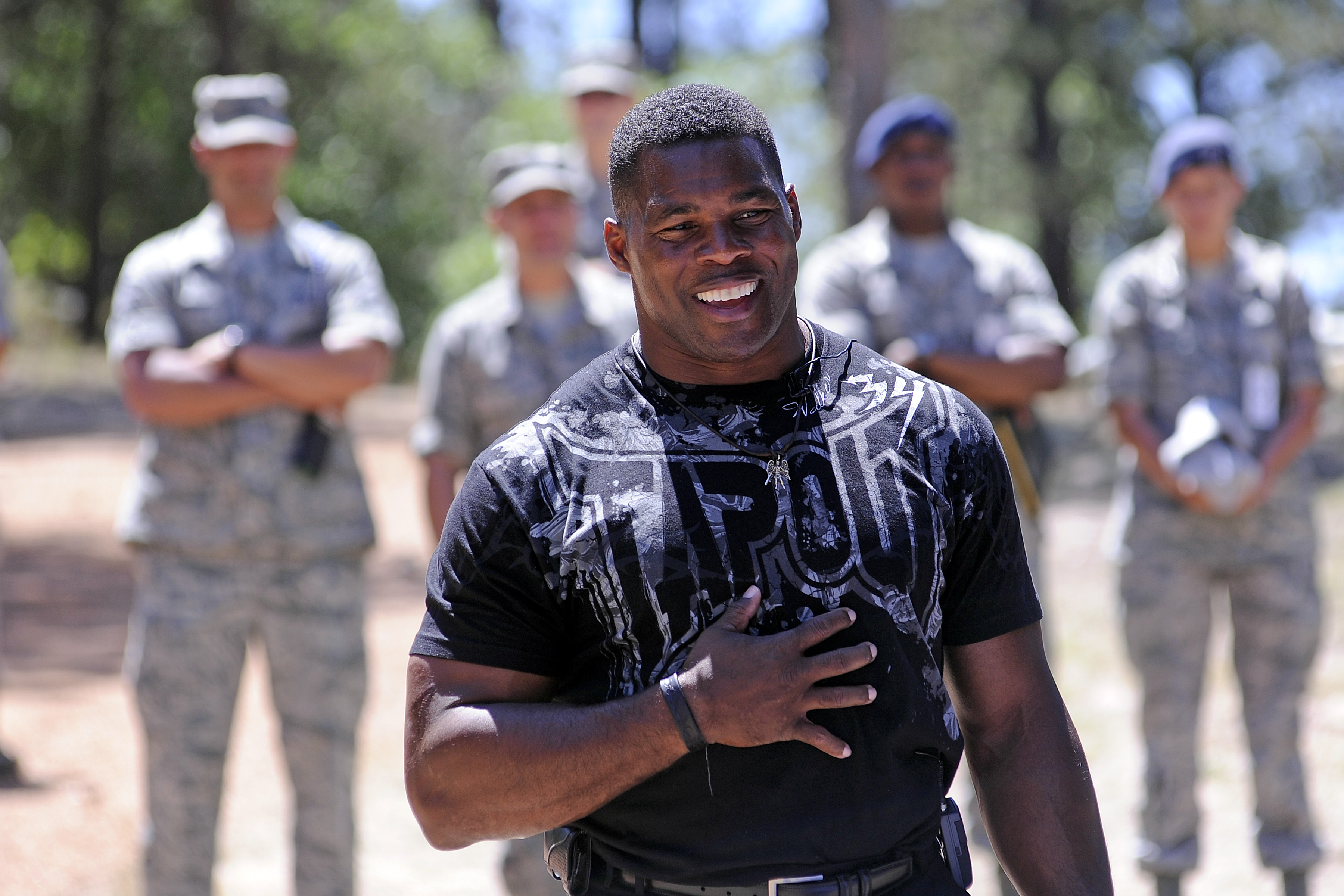The image features an African-American man in the center, smiling and appearing very muscular, captured from the waist up. He is wearing a tight black T-shirt with a graphic design that reads "tap out" in white letters. His short hair is shaved at the sides, and he has a watch on his right wrist. His right hand rests on his chest, possibly slightly above his stomach. Behind him, in a blurred background, stand five soldiers dressed in camouflage fatigues, some wearing camouflage hats and others wearing blue or lighter blue hats. They are positioned in an outdoor setting, likely a forest area, indicated by the visible trees and green foliage. The soldiers' faces and bodies are indistinct, blending into the backdrop of a brown, gravelly or sandy road. The African-American man, who could possibly be a drill instructor or a fitness coach, is the clear focal point of the image.